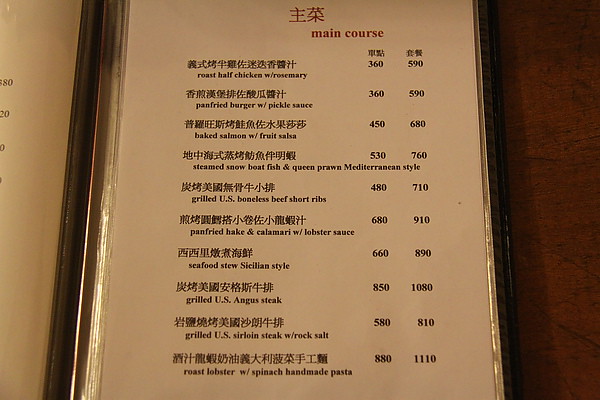The image displays a meticulously designed restaurant menu, presented on a piece of off-white beige paper with an elegant gold trim around its edges. The menu is set in a golden frame, lending a touch of sophistication. Written in both English and Japanese characters, the menu highlights its offerings in a visually appealing manner. The main course items are emphasized in red, starting with:

- Roast Half Chicken with Rosemary: priced at 360 and 590.
- Pan-Fried Burger with Pickle Sauce: priced at 360 and 590.
- Baked Salmon with Fruit Salsa: priced at 450 and 680.
- Steamed Snow Boat Fish and Queen Prawn Mediterranean Style: priced at 530 and 760.
- Grilled U.S. Boneless Beef Short Ribs.
- Pan-Fried Hake and Calamari with Lobster Sauce.
- Seafood Steel Sesamean Style.
- Grilled U.S. Angus Steak.
- Grilled U.S. Sirloin Steak with Rock Salt.
- Roast Lobster with Spinach Handmade Pasta.

Each dish is accompanied by two different price points, reflecting portion sizes or service variations, tailored to suit diverse preferences. The harmonious blend of languages and luxurious design elements enhances the menu's appeal, making it a feast for the eyes as well as the palate.